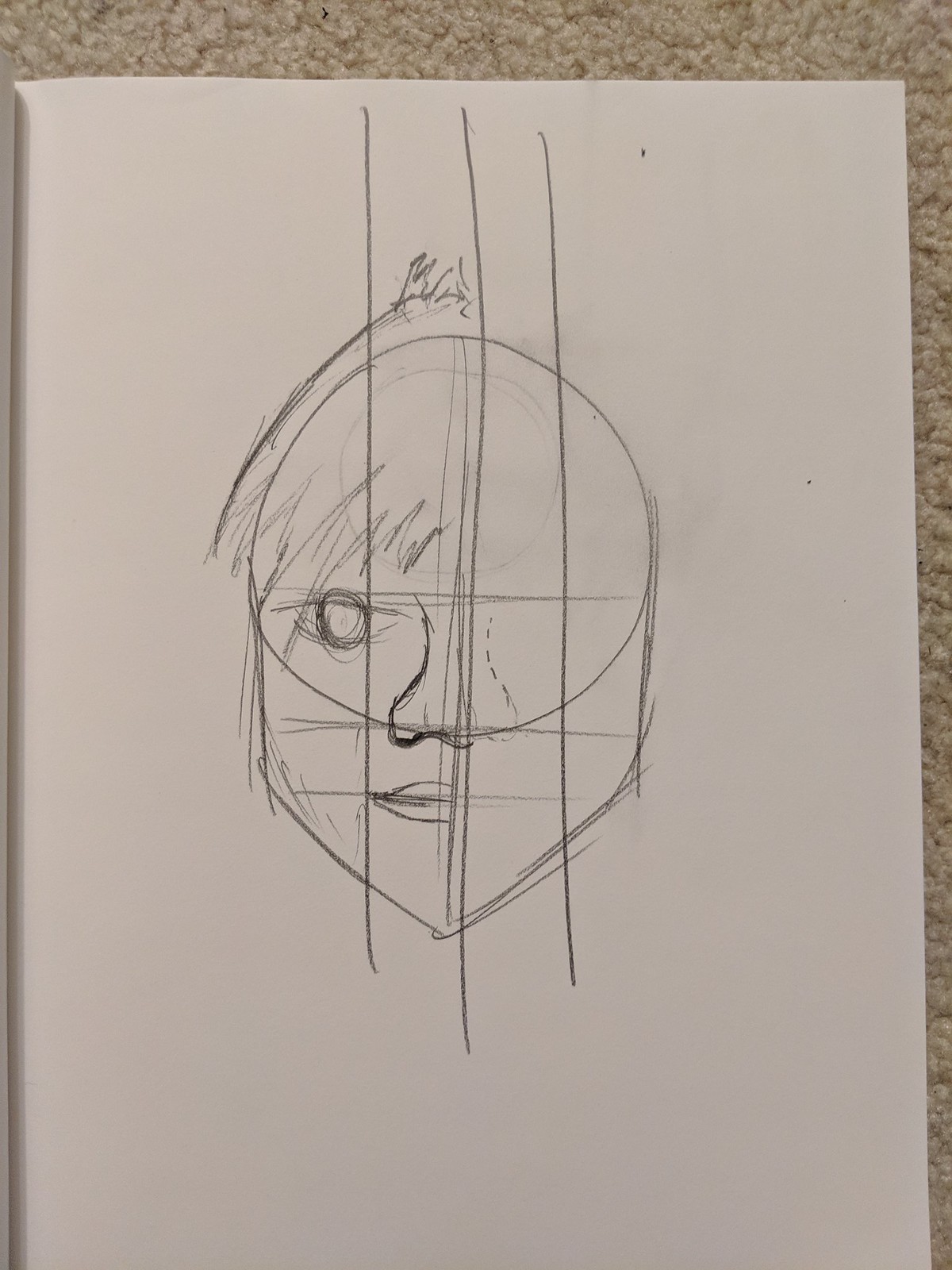This image features an intricate pencil drawing of a human face, carefully positioned atop a piece of white paper resting on a beige, low-pile carpet. The drawing captures a partial visage, focused primarily on the right eye of the subject. The eye is meticulously detailed, standing out as the focal point. The nose is artistically highlighted with a dark shadow on the left side and depicted with a series of dots on the right, adding a unique texture.

The left side of the mouth is clearly defined and solid, contrasting with the absence of the right side, giving the face an unfinished yet compelling look. Short, spiky hair adorns the top left of the head, adding character and framing the top of the face, which sharply tapers into a pointed V-shaped chin.

Notably, the drawing omits the ears and right eye entirely, and no mouth is present on the right side of the face either. Two to three vertical lines run from above the head, through the drawing, and extend below the chin. One line slices directly through the middle of the picture, another passes near the visible eye, and the third delineates where the missing right eye would be. This nuanced and thoughtfully detailed piece evokes a sense of abstract incompletion and artistic exploration.